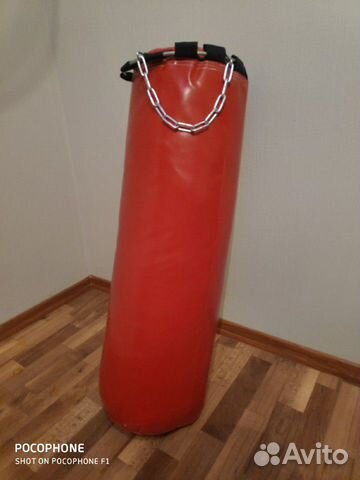The image, which appears to be a photograph or a photorealistic rendering, captures a large, bright red punching bag resting on the floor in the corner of a room. The punching bag, made of glossy leather, is not suspended but instead leans against a white wall. At the top of the bag, black bands secure silver chains and a metal ring, designed for hanging. The floor is a mix of light and dark brown wooden planks, and there is a wooden baseboard at the bottom of the wall. Reflective light on the top of the bag adds a subtle gloss. The text "Pocophone, Shot on Pocophone F1" is visible in small white letters at the bottom left of the image. On the bottom right, semi-transparent white text reads "Avito," accompanied by four circles of varying sizes to the left of the word. This detailed scene emphasizes the prominent red punching bag in a minimalist, well-lit corner setting.